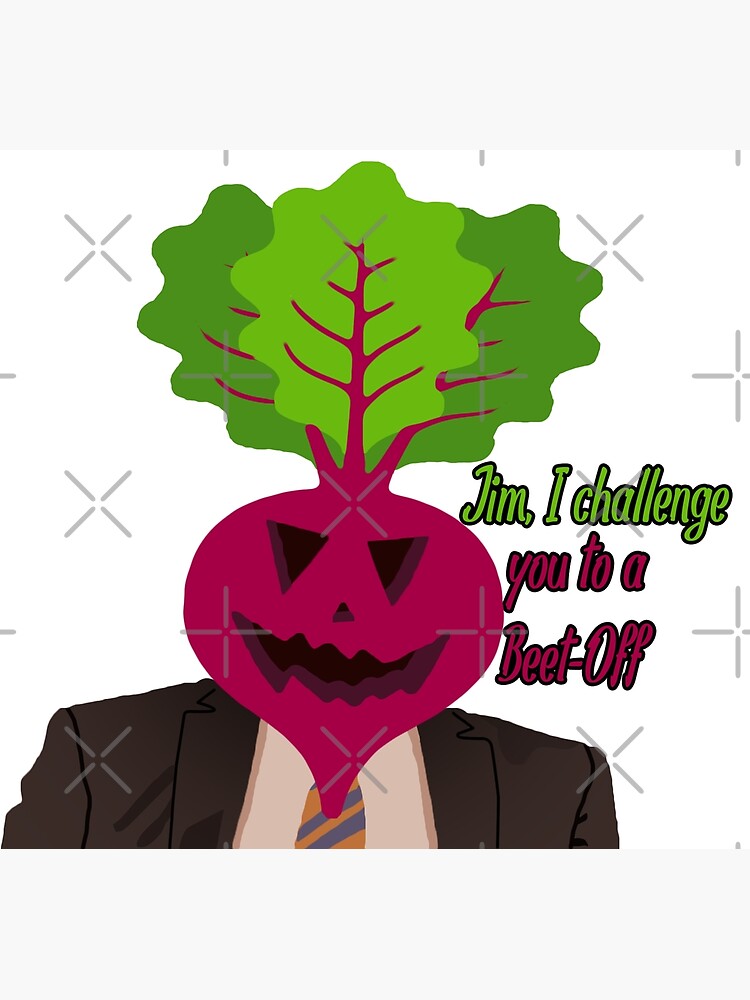This detailed illustration depicts a man in a suit with a beet for a head. The beet, positioned where the man's head should be, is intricately carved like a jack-o'-lantern, featuring downward-pointing triangle eyes, an upward-pointing triangle nose, and a jagged, sinister smile. Green leafy stems sprout from the top, resembling hair. The man is dressed in a dark suit with a striped tie that includes shades of orange and blue. Beside the beet head, the phrase "Jim, I Challenge" is written in green, while "U2A Beat-Off" appears in purple. The background is white, adding to the surreal and peculiar nature of the image.